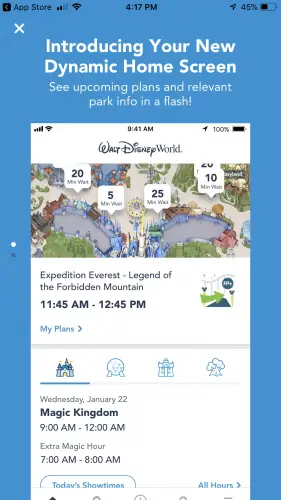"Introducing the new dynamic home screen: A screenshot taken on an iPhone showcases a completely blue background with a small white 'X' icon. In white text, the screen announces upcoming plans and relevant market information. Below, in a smaller white box, details about Walt Disney World are displayed. The text provides specifics about 'Expedition Everest - Legend of the Forbidden Mountain,' along with operational hours. Moreover, events for 'Wednesday, January 22nd' are highlighted, noting that the Magic Kingdom is open from 9 AM to midnight, including an extra magic hour. On the top, several icons allow users to switch views and access showtimes for the day, complete with clickable navigation links."